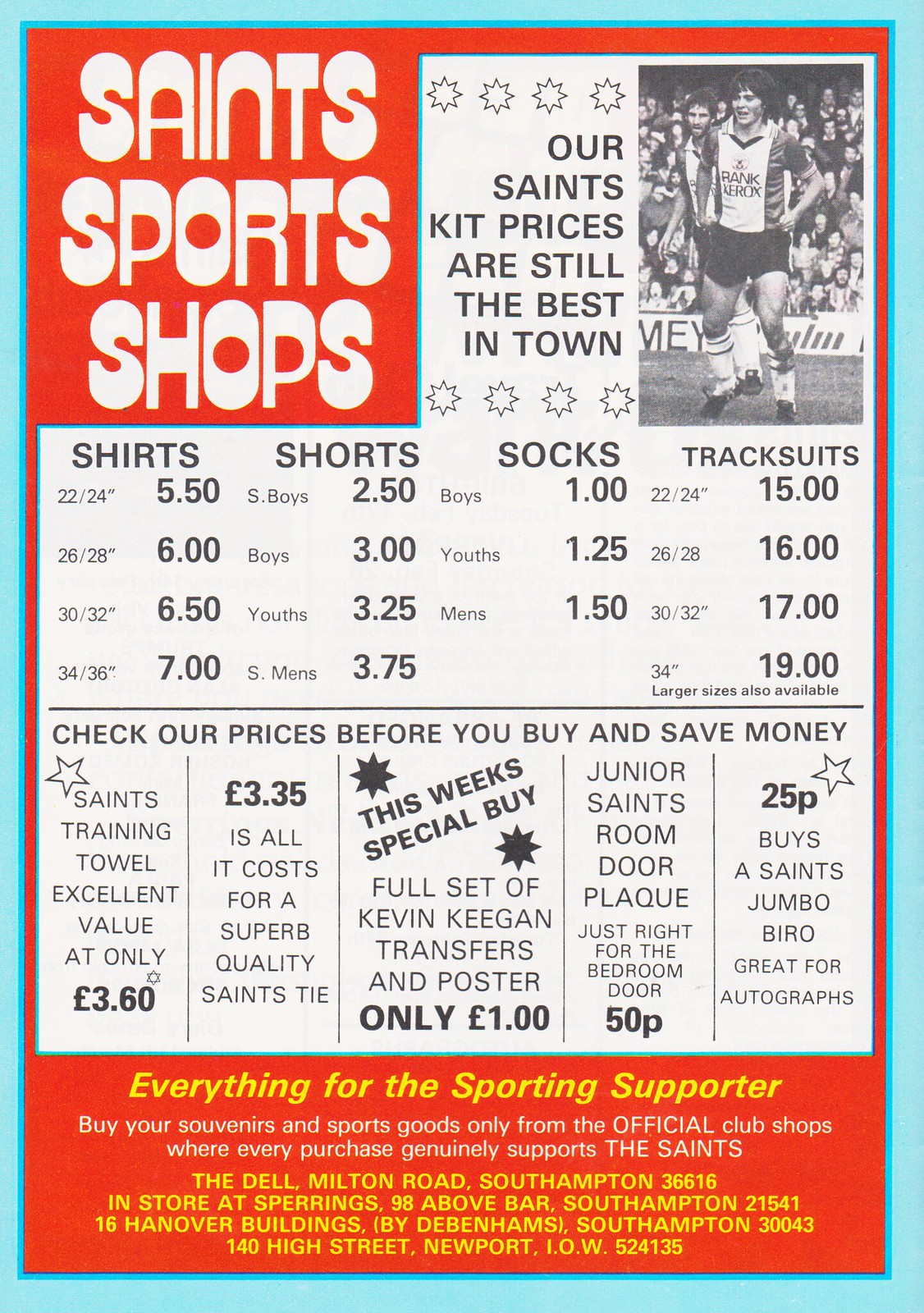The image is a detailed advertisement flyer for Saints Sports Shops, featuring a prominent red background with white, uppercase lettering. In the top left corner, it reads "SAINTS SPORTS AND SHOPS." To the right, a larger white box extends downward, prominently displaying the message, "OUR SAINTS KIT PRICES ARE STILL THE BEST IN TOWN," surrounded by small stars. Adjacent to this, on the top right, is an image of a soccer player in full kit.

Below this central section, the flyer is divided into columns listing prices for various sportswear items: shirts, shorts, socks, and track suits. Shirts are priced between $5.50 and $7.00, shorts range from $2.50 to $3.75, socks are available for $1.00 to $1.50, and track suits are listed from $15.00 to $19.00. Further down, another section urges shoppers to "CHECK OUR PRICES BEFORE YOU BUY AND SAVE MONEY."

The bottom of the flyer features a continuation of the red background with white and yellow text, ensuring the advertisement is visually cohesive and appealing while clearly communicating the message and deals available at Saints Sports Shops.